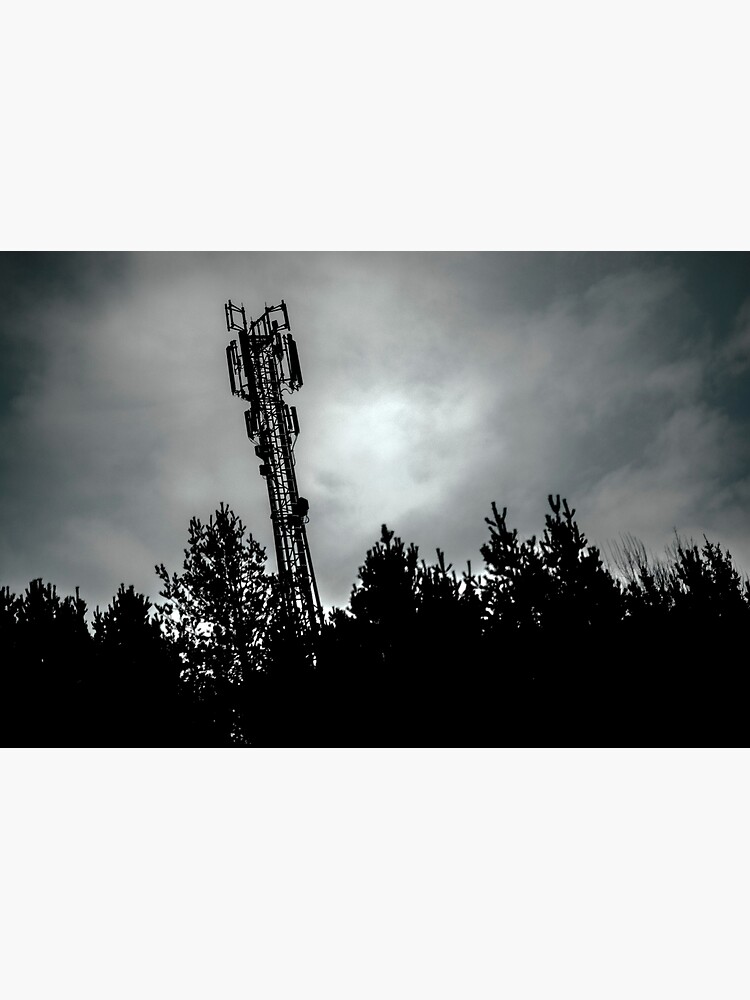The image depicts a nocturnal outdoor scene dominated by a dramatic, overcast sky that ranges in color from deep black and gray to darkish grayish-blue tones. The sky is the most noticeable feature, filled with thick clouds that suggest an impending storm or a moonless night. Below the vast expanse of sky, a forest treeline forms the base of the image, creating a natural frame that contrasts with the artificial elements present.

Slightly to the left and leaning, stands a large metal structure, which appears to be a telephone pole. Its intricate parts and towering height, possibly 20 to 30 stories, give it an imposing presence that hints at its potential function as a conductor of electricity or as part of a launch system for rockets, adding a sense of mystery and scale.

The atmosphere of the scene is one of quiet solitude, out in the open, emphasizing the stark contrast between the man-made metallic structure and the serene, shadowed treeline below. No text features in the image, allowing the viewer to focus entirely on the interplay of natural and industrial elements bathed in the somber hues of the night.